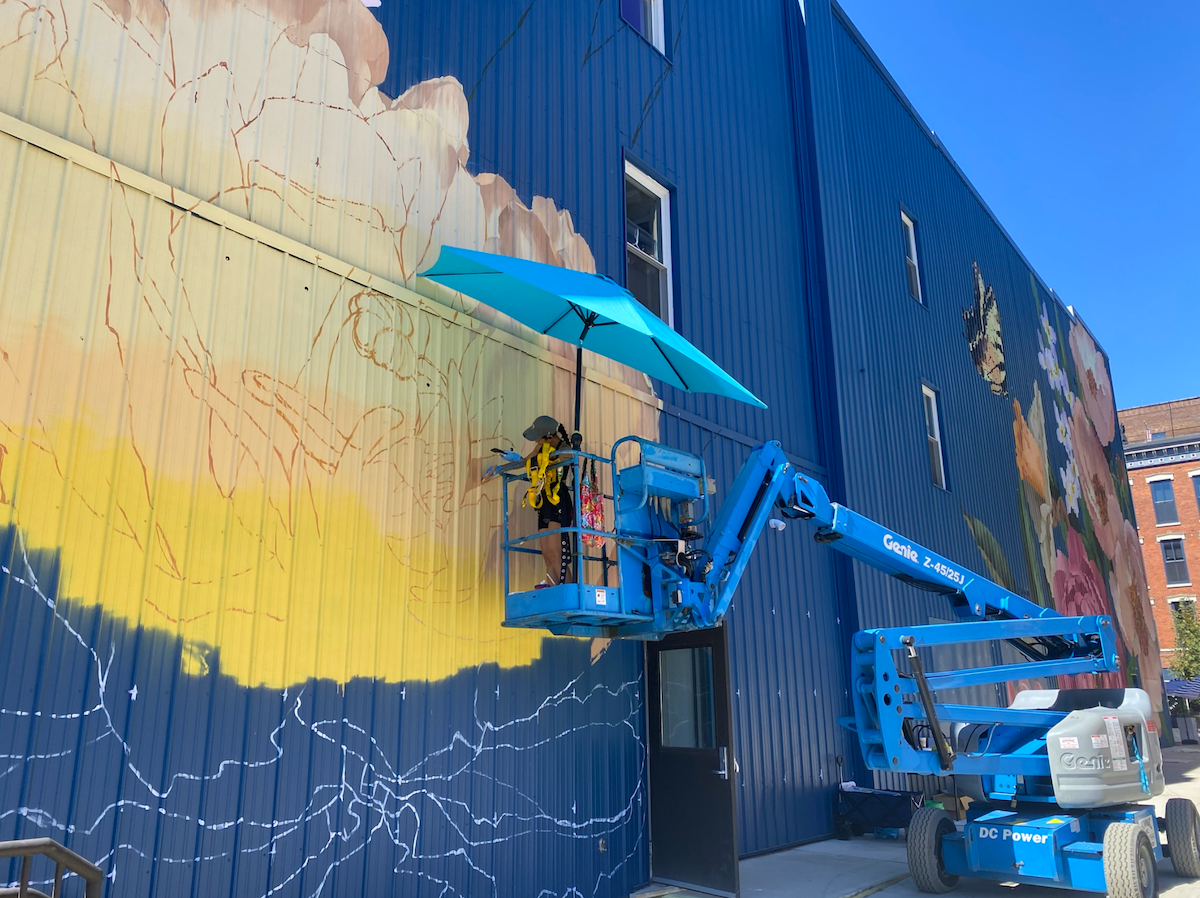The image shows the side of a large, dark navy blue metal warehouse building adorned with a massive, vibrant mural featuring beautiful flowers and a butterfly. A blue crane, equipped with a small platform and a blue umbrella for shade, lifts a woman high up to the building’s side, where she continues her artistic work. She appears to be the same artist who painted the completed mural on one end of the building and is now sketching and filling in a new floral mural on another section. The mural in progress showcases colors like yellow, salmon, and off-white. The scene is set against a flawless blue sky, and in the background, there is a reddish-orange brick building. The details of the mural, the artist's equipment, and the clear blue sky all contribute to the vibrant and dynamic atmosphere of the image.